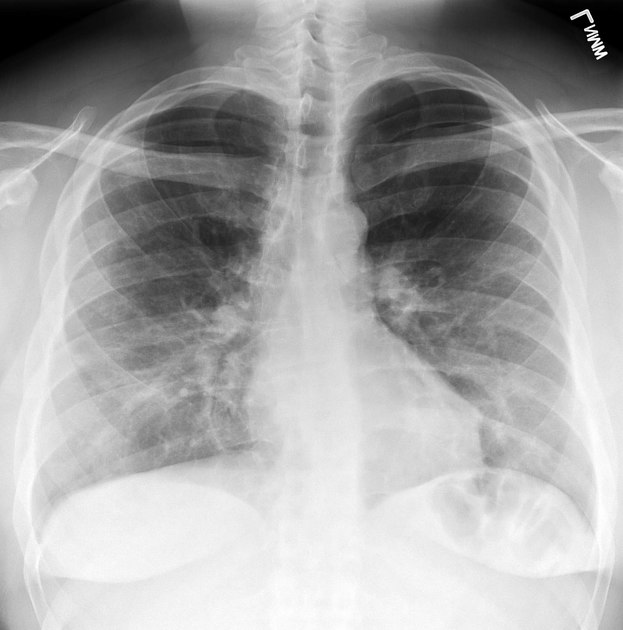This image showcases a chest x-ray, depicted in black and white, with varying depths and shadows indicating different tissues and structures. The perspective appears to be from the front, clearly highlighting the individual's spine running down the center of the image. Prominently visible are the ribcage, shoulder blades, and collar bones, alongside the darker portions representing the lungs and the diaphragm below them. Additionally, there is a notable marking in the upper right corner of the x-ray, possibly text at a 35-degree angle, which might be mirrored or backward. The detailed visualization is typical, depicting a translucent gray color where bones are represented, providing a comprehensive view of the thoracic skeletal and soft tissue anatomy.